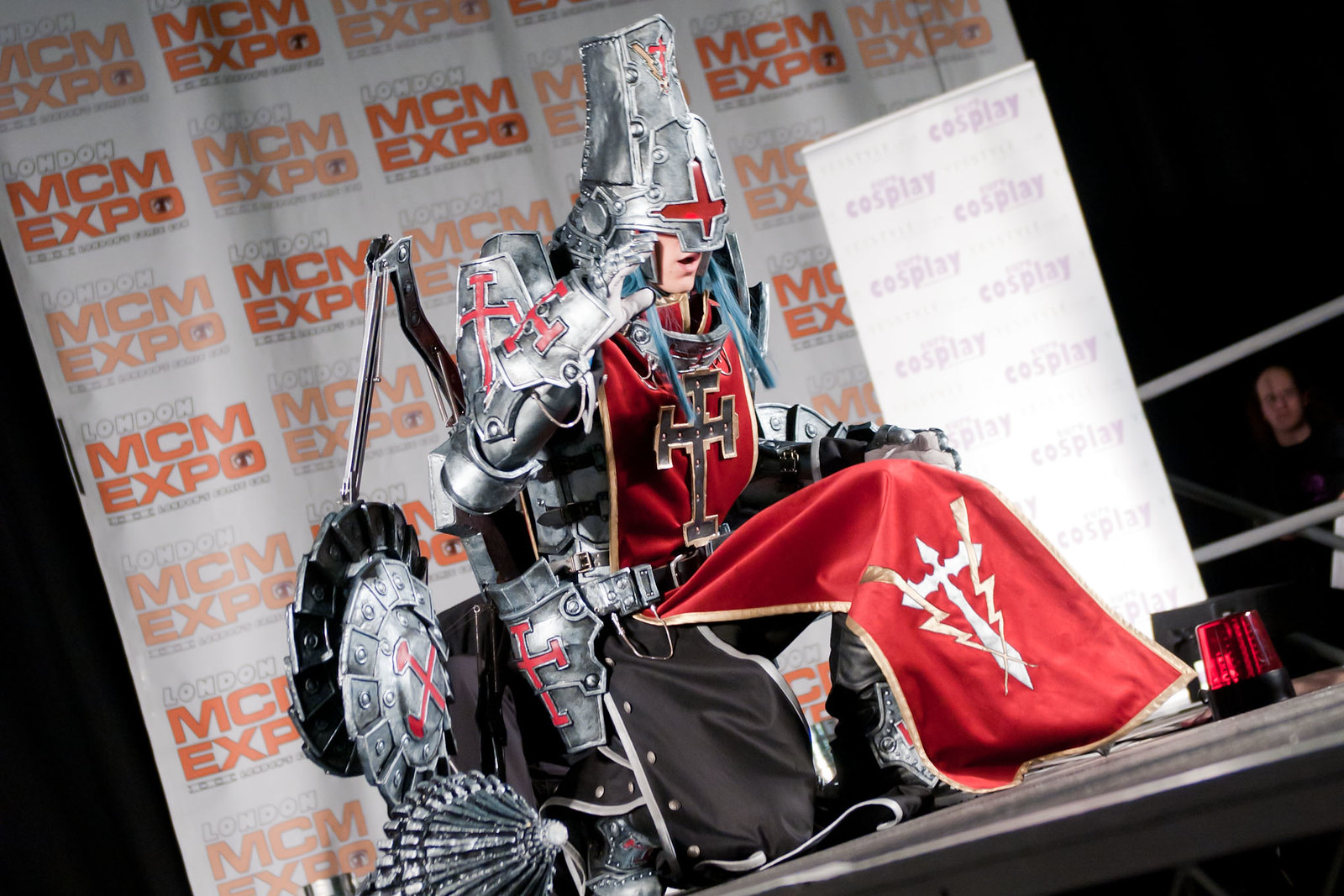The image depicts a man dressed in elaborate medieval knight armor, positioned on a diagonally tilted stage. The knight's costume is composed of intricately detailed dark gray metal armor, complete with a high helmet that hides his eyes and nose, featuring a distinctive red cross in the center. A flowing red and gold satin-like banner adorns his chest, cascading elegantly to the floor. He is kneeling on one knee, with several dark gray metallic weapons and a shield, also emblazoned with a red cross, attached to his attire. The stage's backdrop is adorned with a large white sign displaying a repeating pattern of the words "London MCM Expo" in varying shades of bright and lighter orange. A red light adds a dramatic effect in the bottom right corner of the image.